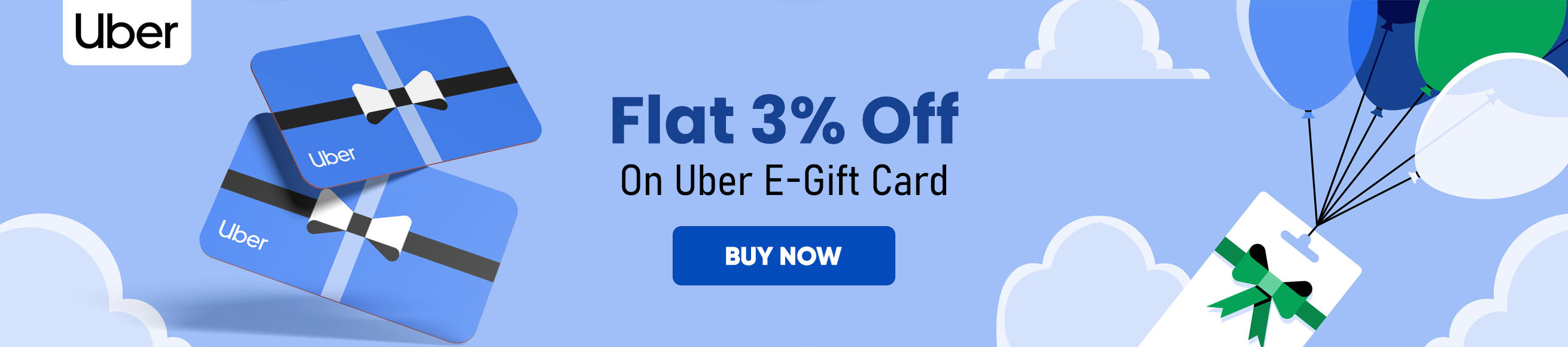This image appears to be a promotional flyer for Uber, set against a light blue periwinkle background. In the top left corner, a small white rectangle prominently features "Uber" in bold black letters. Centrally positioned, the text declares, "Flat 3% Off" with a subheading reading, "on Uber E-Gift Card." Below this, a clickable "Buy Now" button is visible, inviting users to make a purchase. To the left of the central text, two Uber gift cards adorned with decorative ribbons are displayed, enhancing their visual appeal. On the right side, another gift card, tied with a green ribbon, floats skyward, carried by a cluster of colorful balloons. The scene is complemented by several gray and partially white clouds, adding a whimsical, airy touch to the overall design.